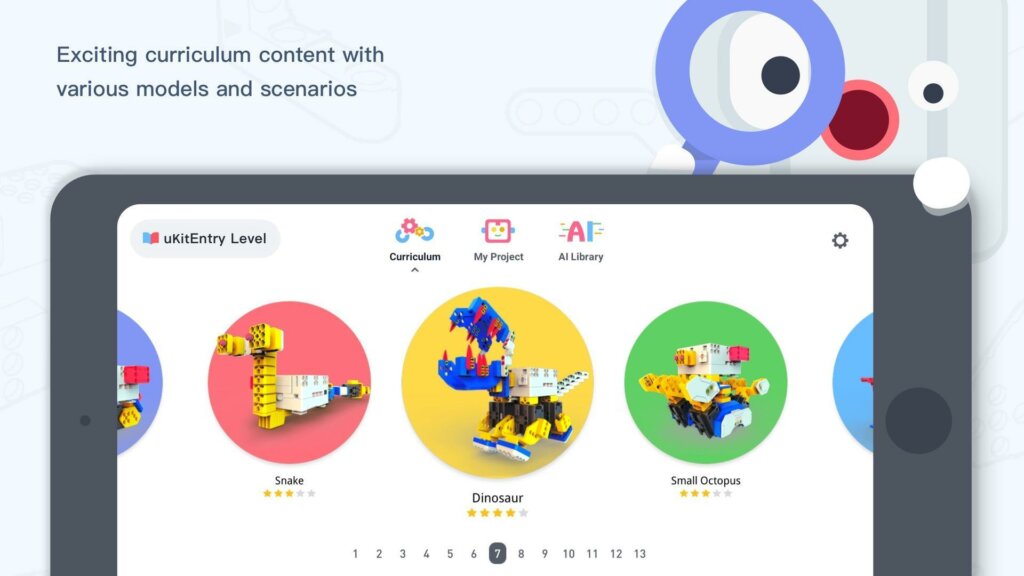This image is an advertisement for the company Ukit, spelled U-K-I-T with a capital "K," which creates products similar to Lego. These products consist of numerous small plastic pieces that children can assemble to create various objects. 

The ad features a light blue background. In the top left corner, there is a piece of dark blue text that reads, "Exciting curriculum content with various models and scenarios." 

On the top right side of the ad, there's a whimsical illustration of a stylized animal. The animal has two large white eyes and a big red mouth, with its right eye peering through a blue magnifying glass directly at the viewer. One of the animal’s paws is placed on the top right corner of an iPad or tablet, which occupies the bottom center of the image.

The screen of the tablet showcases different products that Ukit offers. Displayed are three images: a snake, a dinosaur, and a small octopus. Each product image features the object assembled from Ukit pieces within colored circles—a red circle for the snake, a yellow circle for the dinosaur, and a green circle for the octopus. These images come with links providing detailed information about the products, including purchase options, reviews, and more.

The advertisement seems targeted towards children and looks as though it might be especially appealing for educational purposes, suggesting that teachers or school administrators might consider purchasing these Ukit sets for classroom use.